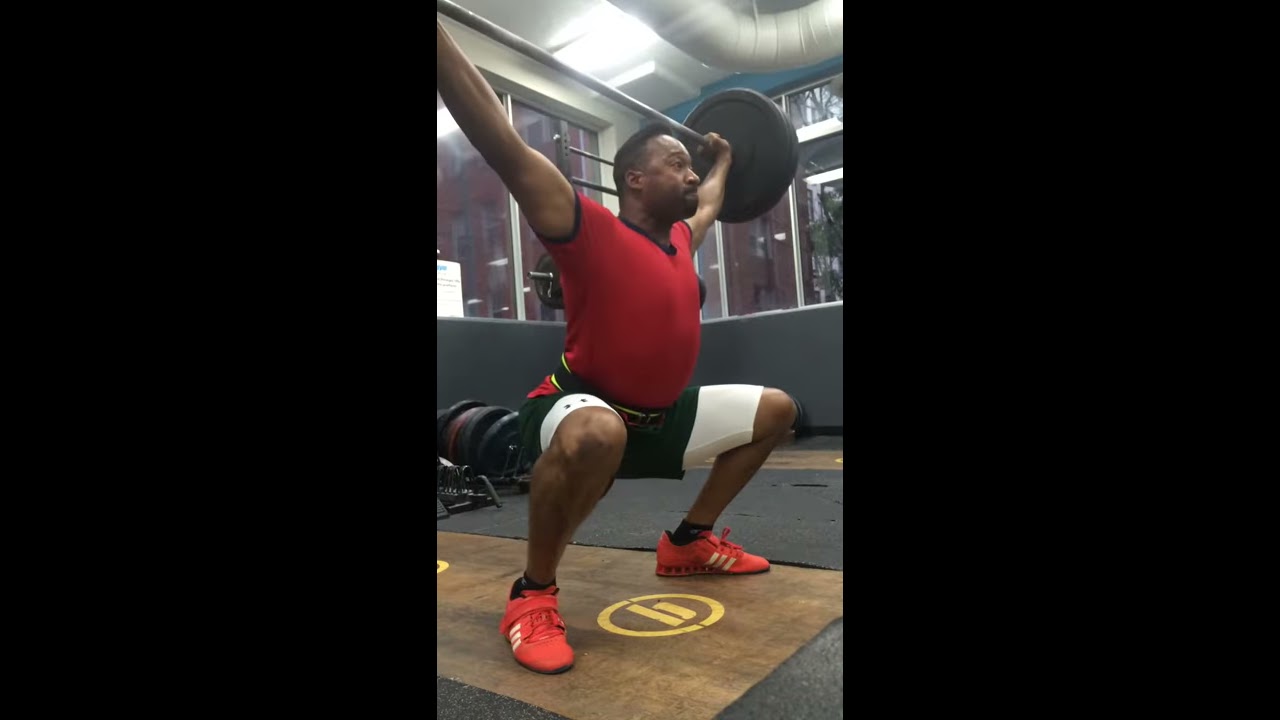In this detailed image, an African-American man is captured in the midst of an intense weightlifting exercise within a gymnasium. He is in a squatting position, thrusting a heavy barbell with weights above his head, seemingly ready to stand up. Dressed in a distinctive red workout shirt with black outlines at the edges, he also wears black shorts over white compression sleeves that extend to his knees, and completes his outfit with red sneakers featuring yellow stripes. A black and yellow lifting belt is cinched around his waist for additional support. The setting is a gym's corner, evident from the wooden floor marked with a yellow circle emblem underneath him, and racks of barbells and weights stacked in the background. The man’s strained expression underscores the effort involved in this vigorous weight training session.